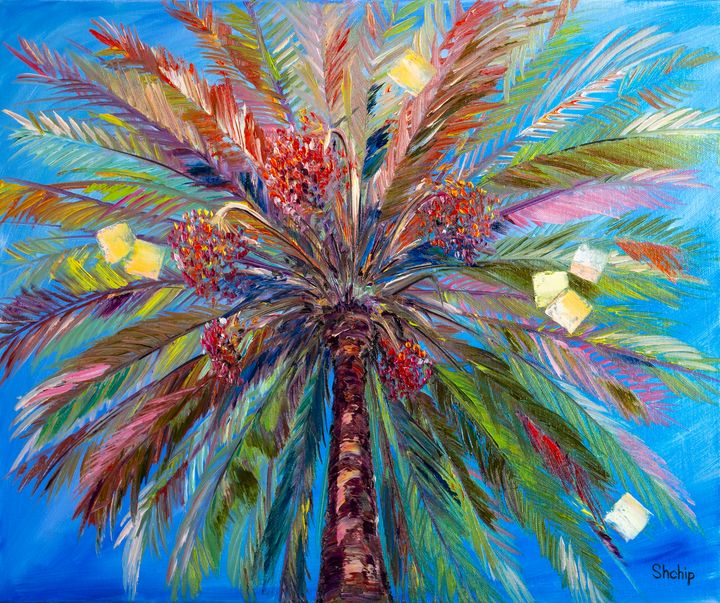The image showcases a detailed drawing or painting of a tall palm tree, centrally positioned against a gradient blue sky that darkens near the bottom. The palm tree features traditional brown bark on its lower section, with palm fronds fanning out in every direction above—a mix of green, red, yellow, and surprisingly, pink hues, adding a burst of unexpected color. Some of the fronds are solid green at the bottom. The tree also bears five bunches of grapes that hang down prominently, suggesting that it could be a date palm. The overall picture is highly colorful and meticulously created, possibly with colored pencils, and is described as a visually pleasing piece that makes for a good place to pause and admire for its vibrant and unique details.